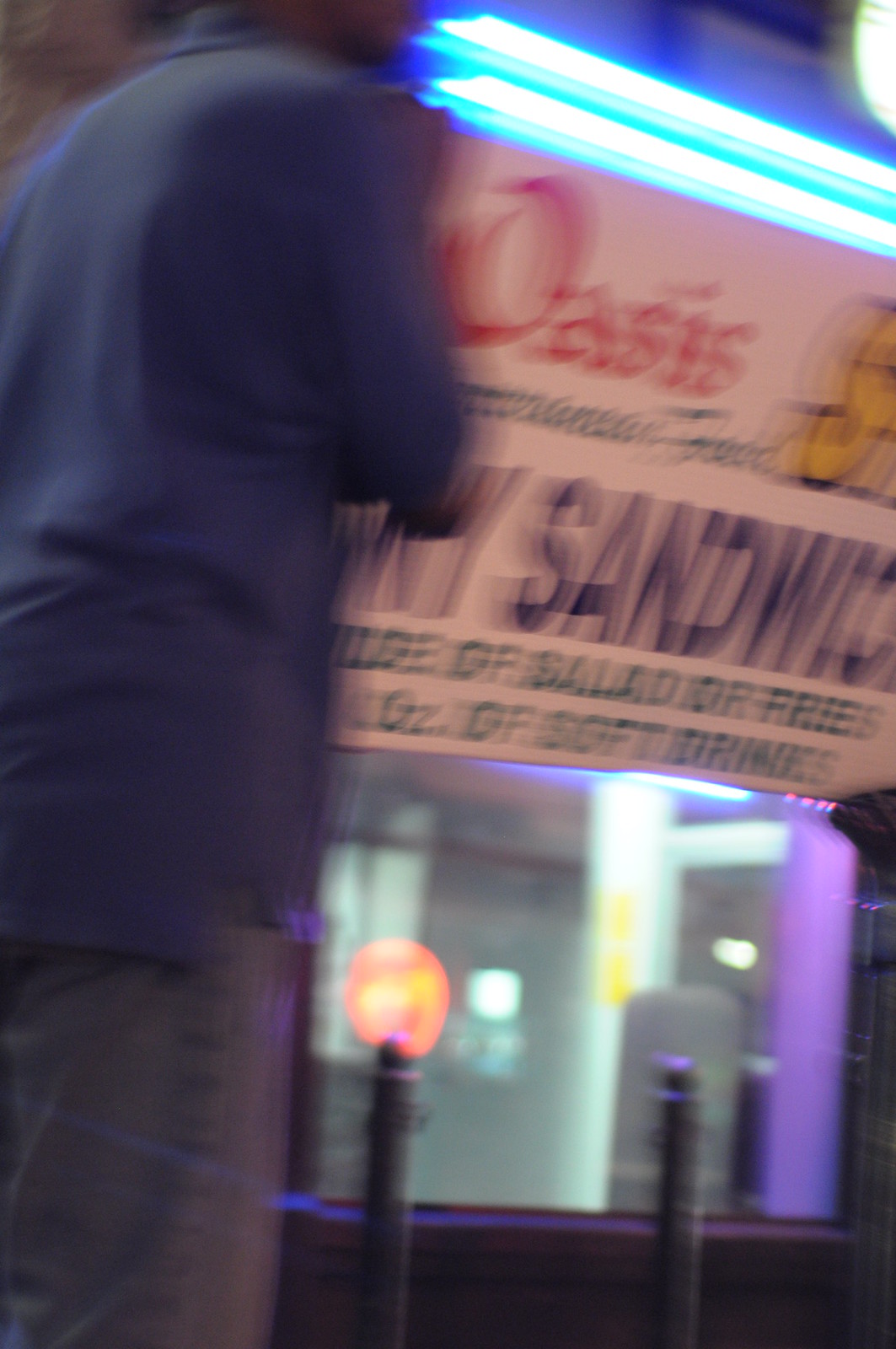This is a blurry, close-up photograph taken at night of a sandwich shop named Oasis. The sign prominently displays "Oasis" in red lettering, with "NY Sandwich" in blue lettering beneath it, followed by "Free Soft Drink" in green letters. The sign is flanked by a bluish LED light and possibly reflects light from across the street. Central to the image is a glass or plexiglass booth, partitioning the ordering area, which also shows some white beams or pillars inside. Standing in front of the booth is an individual on the left side of the image, wearing a navy blue long-sleeve shirt and light blue jeans, possibly in line or waiting for their sandwich. The photograph also displays small gray circular posts that seem to guide the queue.